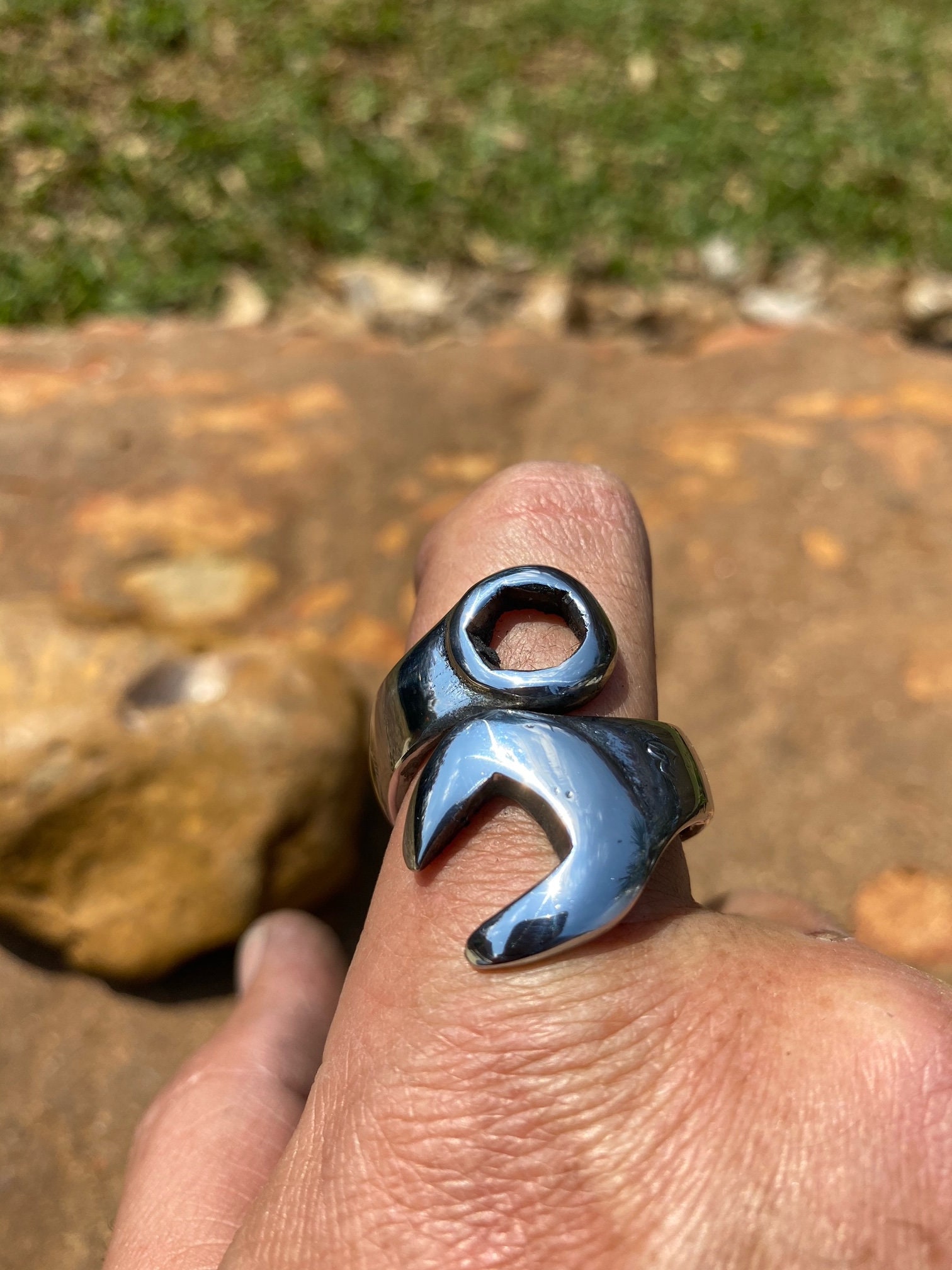In this bright, sunlit outdoor scene, a White Caucasian man's hand prominently displays a unique silver ring on his index finger. The focus of the picture is on his hand, where the other fingers are folded down, and his thumb is visible to the side. The silver ring itself is intriguingly shaped like a wrench, cleverly designed to wrap around his finger with the head and tail of the wrench meeting seamlessly. The background of the image is intentionally blurred but reveals a natural setting with a dirt-covered ground dominating the lower three quarters of the frame. A large boulder is positioned to the left, with smaller rocks scattered around it. At the upper edge of the photograph, a lush grass area can be seen, indicating the person might be walking on a trail. The abundant natural light suggests the photo was taken on a bright, sunny day.